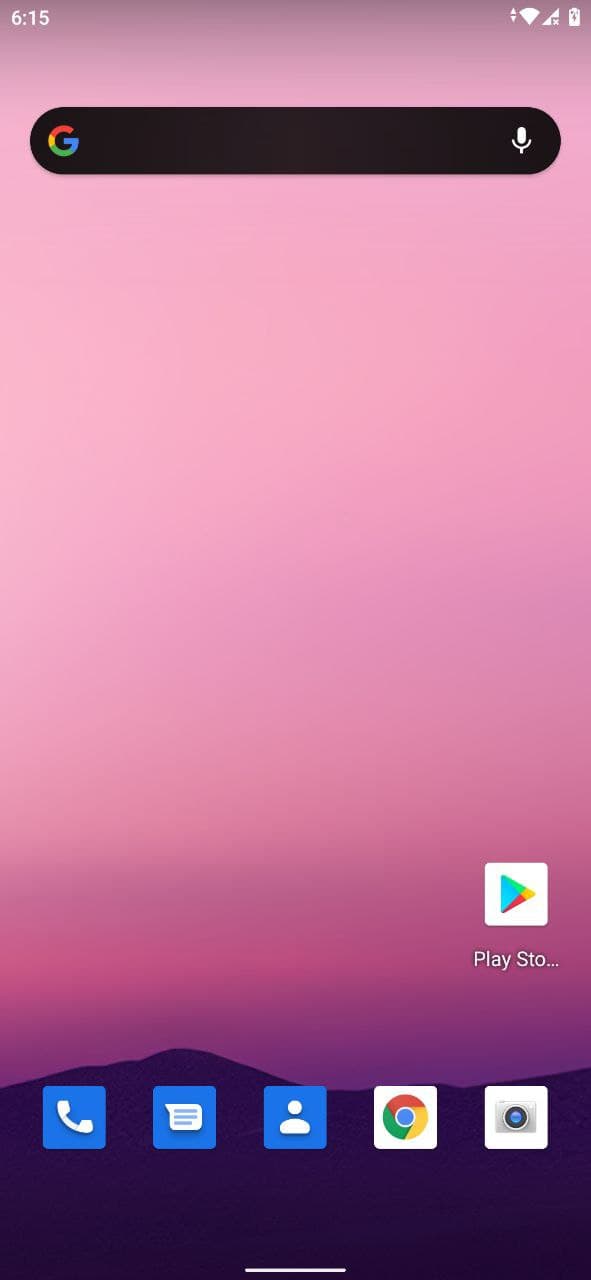The screenshot captures the home screen of an Android phone, featuring a soft, ethereal background that fades from pink to light purple, evoking the colors of a dreamy sky. The serene background is juxtaposed with the silhouette of dark, jagged mountains lining the bottom of the screen, creating a striking visual contrast.

Centered at the top is a Google search bar, complete with a microphone icon on the right for voice-enabled searches. This functional element allows users to either type or speak their queries. The main screen is notably uncluttered, devoid of widgets or additional app icons, emphasizing simplicity and ease of navigation.

Positioned along the bottom of the screen are six app icons. Five of these apps are lined up directly at the bottom: Chrome, Camera, Phone, and Text Messages. Slightly elevated from this row is the Play Store icon, set apart from the others, making it a focal point for quick access to the app marketplace.